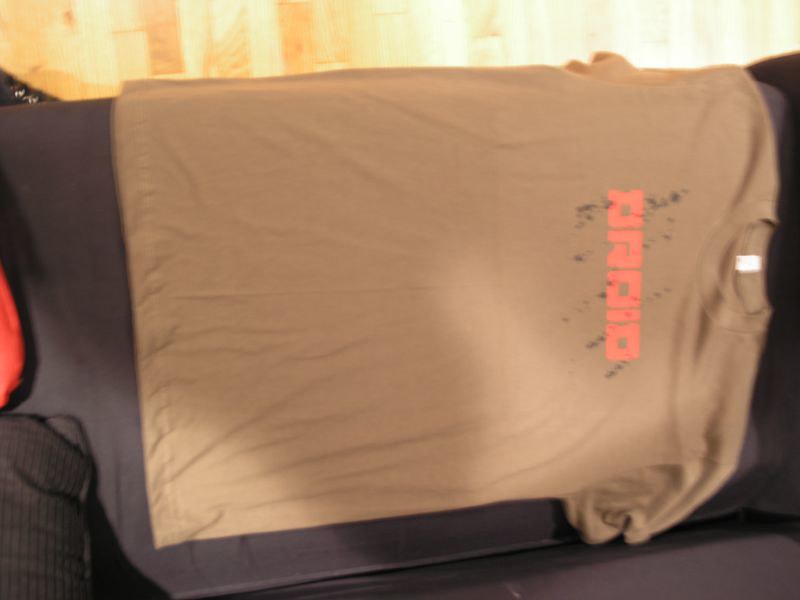In this horizontally oriented photograph, a brown t-shirt is prominently displayed, draped over what appears to be a pillow, though it might also be the end of a couch. The t-shirt is rotated 90 degrees clockwise from our perspective, giving us a side view. It is slightly wrinkled and shows signs of wear, with colors that appear somewhat faded. The shirt has short sleeves and is adorned with red, science fiction-inspired lettering that reads "DROID," possibly a reference to Star Wars. Intricately, the letters are adorned with brown lines running through them. There is a hint of another object on the far left, tinged with orange, suggesting either another piece of clothing or another part of the pillow. Above the t-shirt, a yellow area hints at reflected light, likely from a nearby wall or the floor. The composition of the scene suggests a casual setting, probably involving a piece of furniture like a couch.